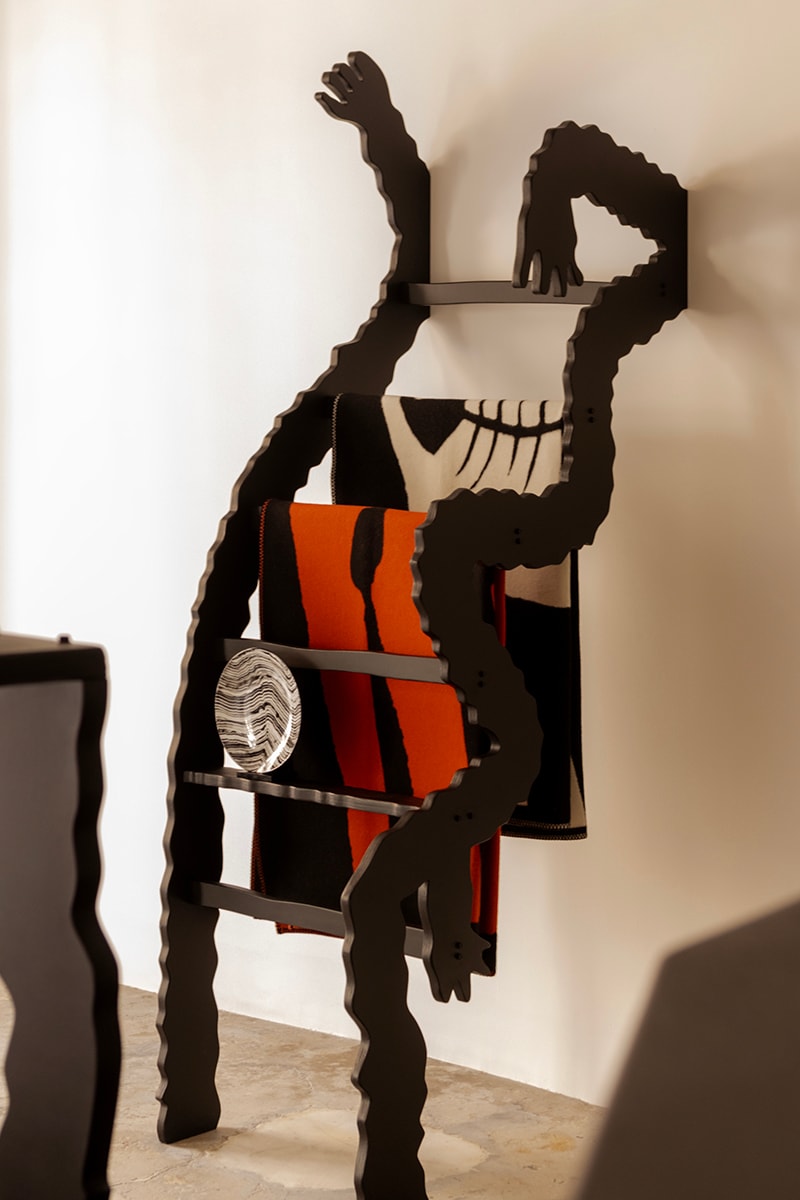The image features an abstract and unique art installation resembling a ladder or a display shelf, leaning against an off-white, eggshell-colored wall. The floor beneath it contrasts with a beige, yellowish, marble-like appearance. The structure, possibly wooden or metal, has elongated, bumpy arms on either side, resembling hands at the top, adding an avant-garde touch to the piece. Five rungs connect the sides, with two displaying textiles: one in orange and black stripes, the other in white and black stripes, possibly Indian-style blankets. A shiny white plate with wavy black lines rests between two of the lower rungs. In the lower corners of the image, other brown wooden structures are partially visible, hinting at matching decor but remaining indistinct.